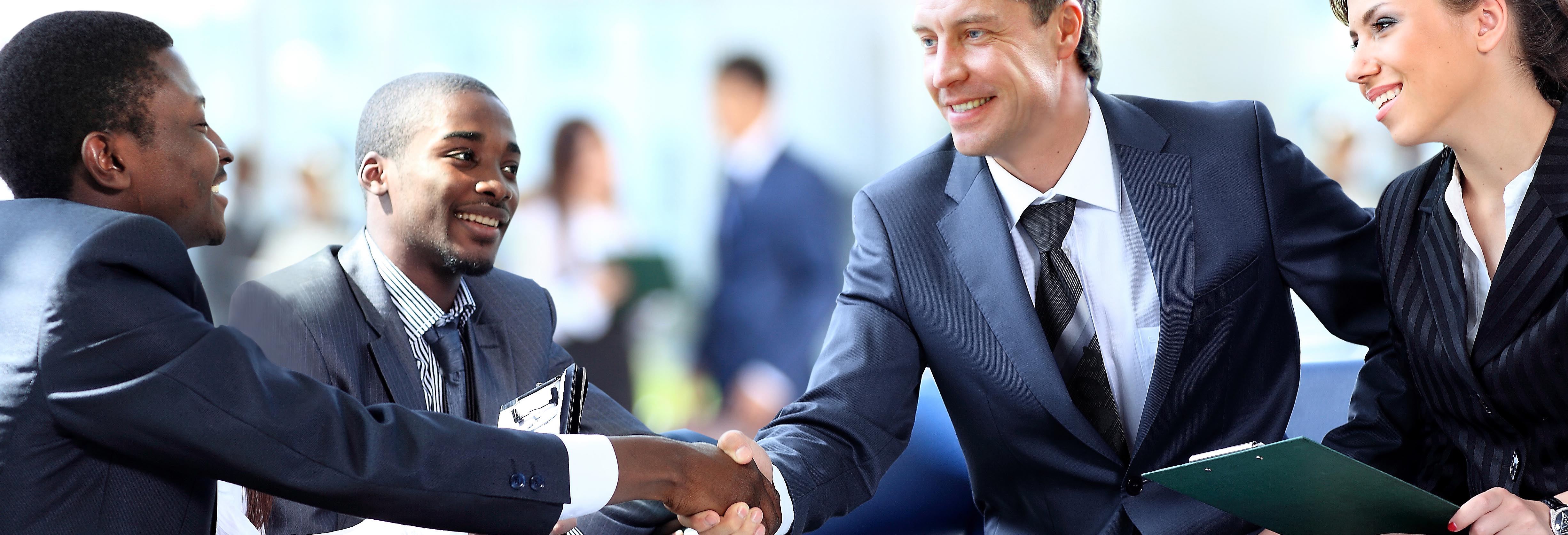This image captures a staged business meeting designed for a stock photograph, featuring four main individuals in sharp focus against a blurred background of indistinct figures. Central to the scene are two men in blue suits shaking hands: a white man on the right who faces the camera, and a Black man on the left shown in a side profile. Both men wear white dress shirts and ties, exuding professionalism. Next to the white man on the right is a white woman in a black striped blazer with a white shirt underneath, holding a green clipboard and smiling warmly. The Black man on the left is accompanied by another Black man, also in a suit and tie, who is smiling and looking towards the two men shaking hands. The background, though populated, remains indistinct and out of focus, emphasizing the interaction in the foreground. This could be a promotional image for a firm, depicting a successful and amicable business meeting.